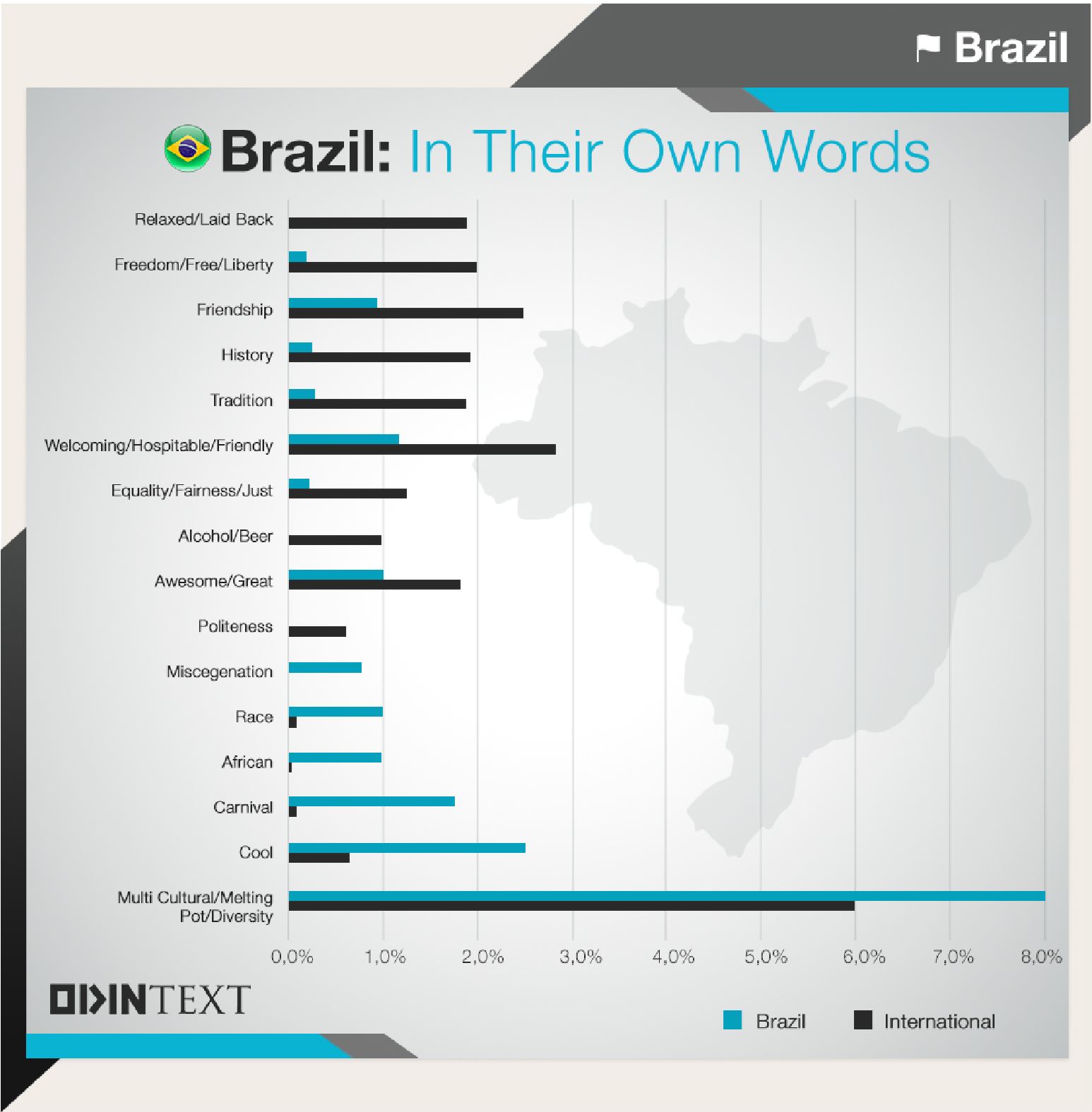In this screenshot, the background features a diagonal division with white in the upper left, transitioning to gray in the center, and returning to white in the lower portion. At the center of the image is a prominent gray box displaying the word "Brazil" in large, bold, black text. To the right of "Brazil," there's a blue text banner and a gray and blue banner in the upper right corner.

The detailed vertical list reads as follows, top to bottom: "Relaxed," "Laid back," "Freedom," "Free," "Liberty," "Friendship," "History," "Tradition," "Welcoming," "Hospitable," "Friendly," "Equality," "Fairness," "And just," "Alcohol," "Beer," "Awesome," "Great," "Politeness," "Miscegenation," "Race," "African," "Carnival," "Cool," "Multicultural," "Melting Pot," and "Diversity."

On the left side of the image, a graph is depicted starting at zero in the lower left corner, with percentage increments from 1% to 8%. The key for the graph includes a blue box labeled "Brazil" and a black box labeled "International."